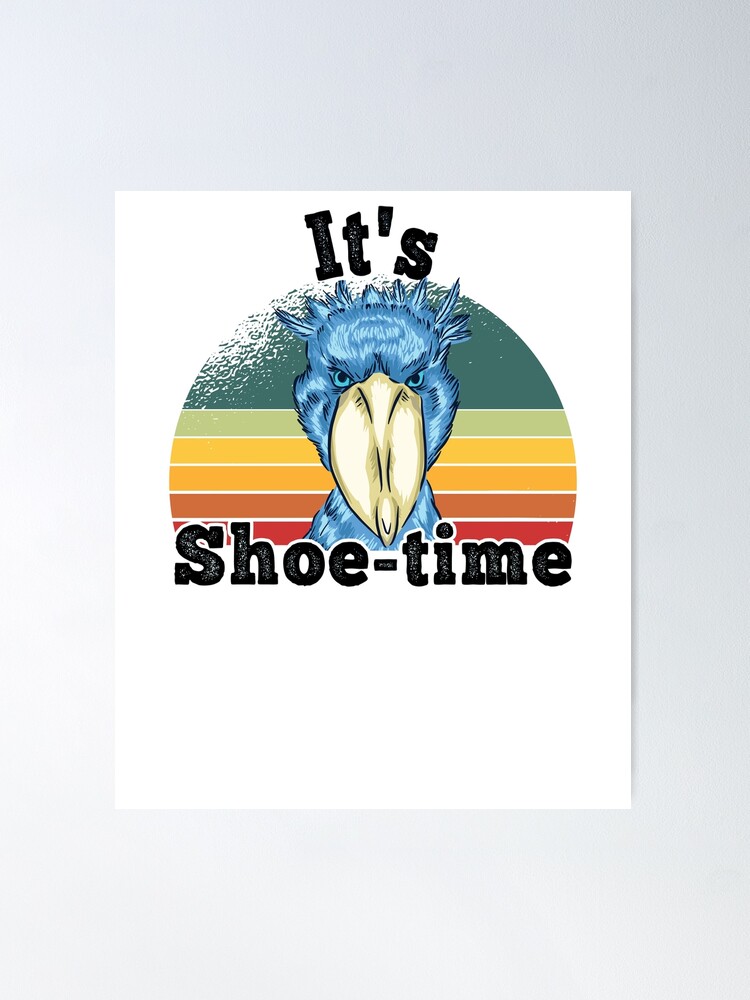The image features a vibrant and detailed illustration set against a stark white background. Central to the design is a striking blue bird with penetrating blue eyes and a large pale yellow beak. The bird, which appears to be looking directly at the viewer, is positioned in front of a semicircle adorned with horizontal stripes in an array of colors: starting from the top with dark green speckled with white, followed by pastel light green, yellow, orange, dark orange, and red. The stripes add a dynamic, energetic background to the bird’s portrait. Surrounding the bird are the bold black words "It's Shoe Time," with "It's" placed above the bird and "Shoe Time" below, slightly faded towards the top, giving the text a slightly worn yet charming appearance. The overall composition, featuring a vivid and clear logo-like illustration, creates a playful and engaging visual, reminiscent of a promotional or branding graphic.